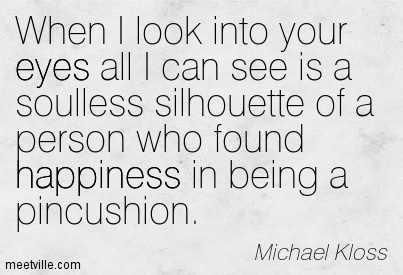The image depicts a quote over a subtly textured background that suggests a marble or light blue stone appearance. The quote is formatted in six lines with key words bolded for emphasis and reads: “When I look into your eyes, all I can see is a soulless silhouette of a person who found happiness in being a pincushion.” The word "eyes" and "happiness" are highlighted in bold. The quote is attributed to Michael Kloss, whose name appears in a thin black font on the lower right corner of the image. On the bottom left corner, there is a website link to meetville.com, the service that likely created the image.